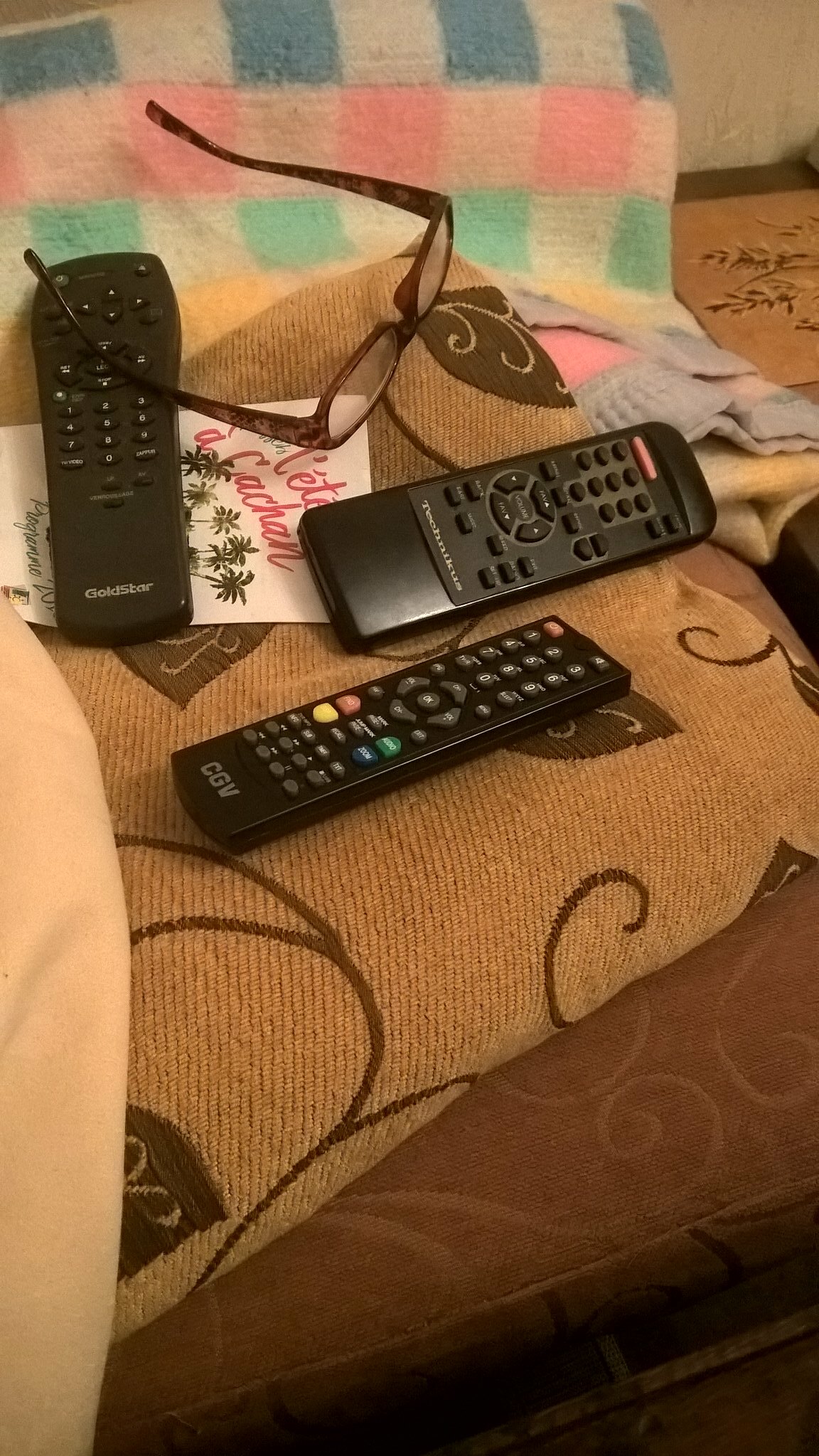This indoor photograph captures a detailed, zoomed-in view of a light brown sofa with intricate chocolate brown designs, presumably located in a living room. On the sofa lies a pile of blankets, over which three black TV remotes are situated. The leftmost remote features black buttons with white symbols. Adjacent to it on the right is another black remote, distinguished by a light red button at its top. The far-right remote stands out with grey buttons, white number and symbol inscriptions, and additional variably colored buttons: red, yellow, green, and blue, with another red button positioned in the top left corner and the letters CGV at its bottom. Nestled amongst these remotes is a holiday card or flyer, partly covered by a pair of glasses whose arm is draped over one of the remotes, infusing a sense of lived-in comfort and everyday technology.